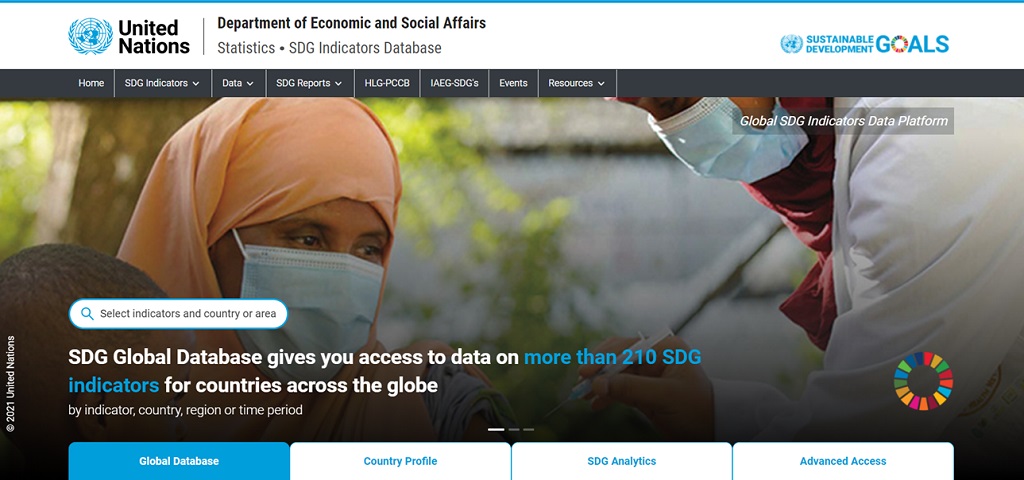This image features a United Nations web page dedicated to the Sustainable Development Goals (SDGs). Displayed prominently in the upper left corner is the United Nations logo, accompanied by the "United Nations" text. Beneath this, the page titles include "Department of Economic and Social Affairs" and "Statistics SDG Indicators Database." In the upper right corner, an eye-catching blue text reads "Sustainable Development Goals."

The navigation menu below includes links labeled: "Home," "SDG Indicators Data," "SDG Reports," "HLG-PCCB," "IAEG-SDGS," and "Events and Resources." Dominating the center of the page is a large image extending nearly the entire width. The image portrays a scene that appears to depict a woman with her identity not clearly discernible; she is wearing a turban and a white face mask and is seated. In front of her stands a figure, presumably a doctor, dressed in a white coat and also wearing a mask, with their face partially obscured. The doctor seems to be administering a vaccine, indicated by the needle poised near the patient's shoulder.

Below this poignant image is a section titled "Select Indicators in Country or Area," which highlights the SDG Global Database. This database provides users with access to data on over 210 SDG indicators, offering insights by country, region, or specific time periods.